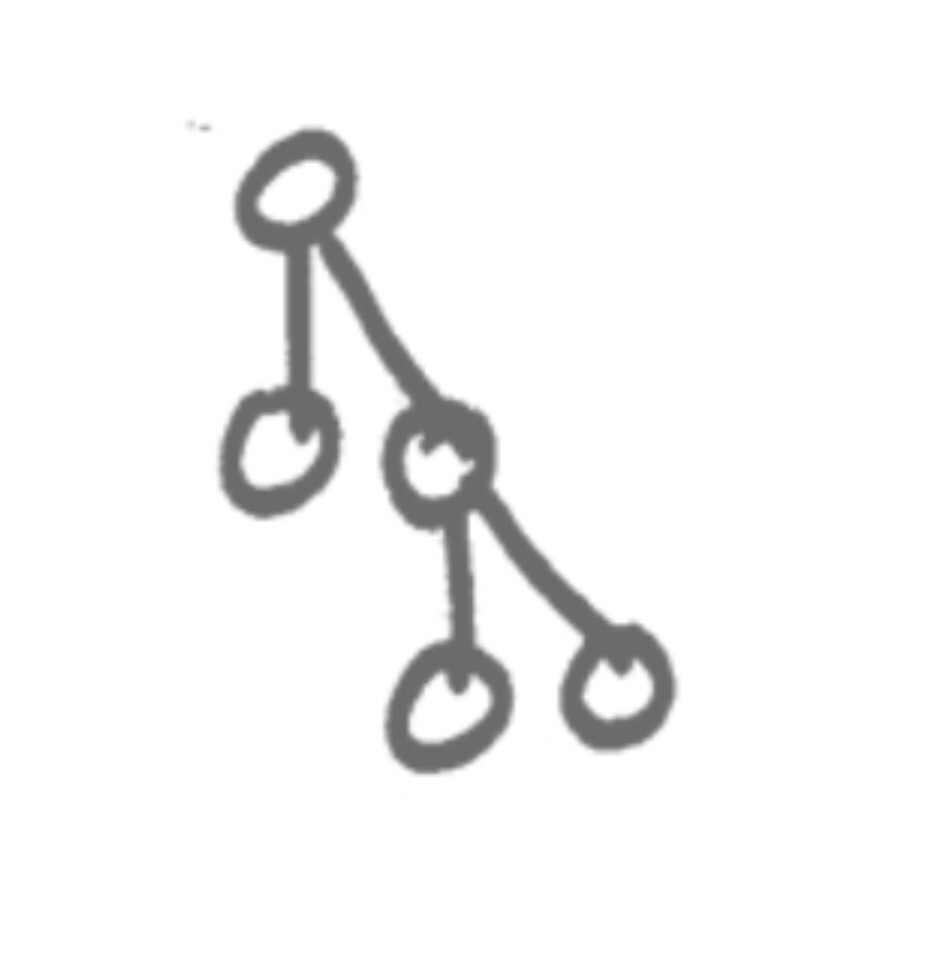A close-up, indoor color photograph captures a hand-drawn diagram on a pristine white background. The focal point is a network of interconnected circles and thick gray lines, illustrated in a rough, freehand style. In the upper left corner, we observe a prominent circle with a vertical line extending downward to another circle positioned centrally in the image. From the top circle, a diagonal line stretches towards the upper right corner, terminating at another circle situated roughly an inch or two downward. An additional segment from this circle extends diagonally downward to yet another circle in the lower right corner.

The central circle features a line radiating straight downwards, connecting to a subsequent circle below it. This creates a mirrored, repeating pattern that anchors the right side of the drawing. Notably, all the lines extend slightly into the interiors of the circles rather than stopping at their edges, suggesting a deliberate stylistic choice. The absence of any words, text, or print directs the viewer's focus solely on the geometric arrangement. This simple yet intriguing sketch resembles a molecular or biological diagram, hinting at possible scientific or educational intent.